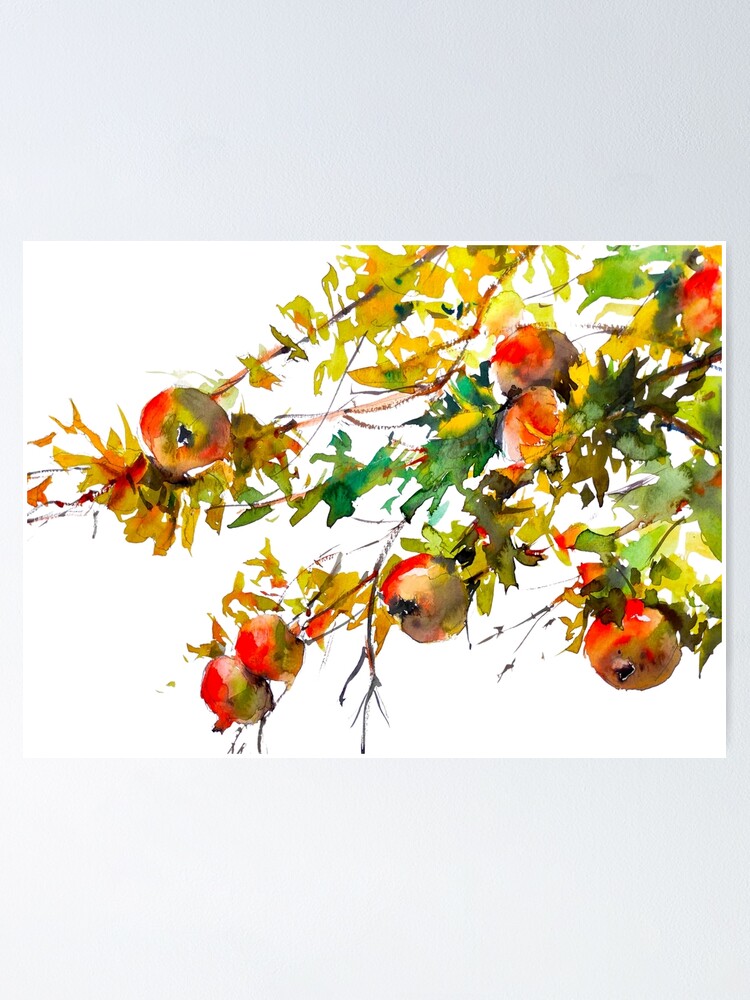This painting, set against a pure white background, intricately depicts an apple tree's branches adorned with a variety of colorful leaves and fruit. Branches extend across the canvas, originating from the upper right-hand corner and gracefully cascading towards the bottom left. The foliage is a vibrant mix of green, yellow, gold, and occasional hints of red and brown leaves. Each branch cradles several pieces of fruit, primarily appearing as apples, but with some variations making them resemble other potential fruits like pomegranates or oranges. The apples themselves are primarily a striking mix of reddish-orange, yellow, and green, with some appearing more ripe than others. The painting style is loose yet detailed, capturing the essence of the leaves and fruit without rigid precision, creating a visually rich and dynamic composition that's both bright and inviting.